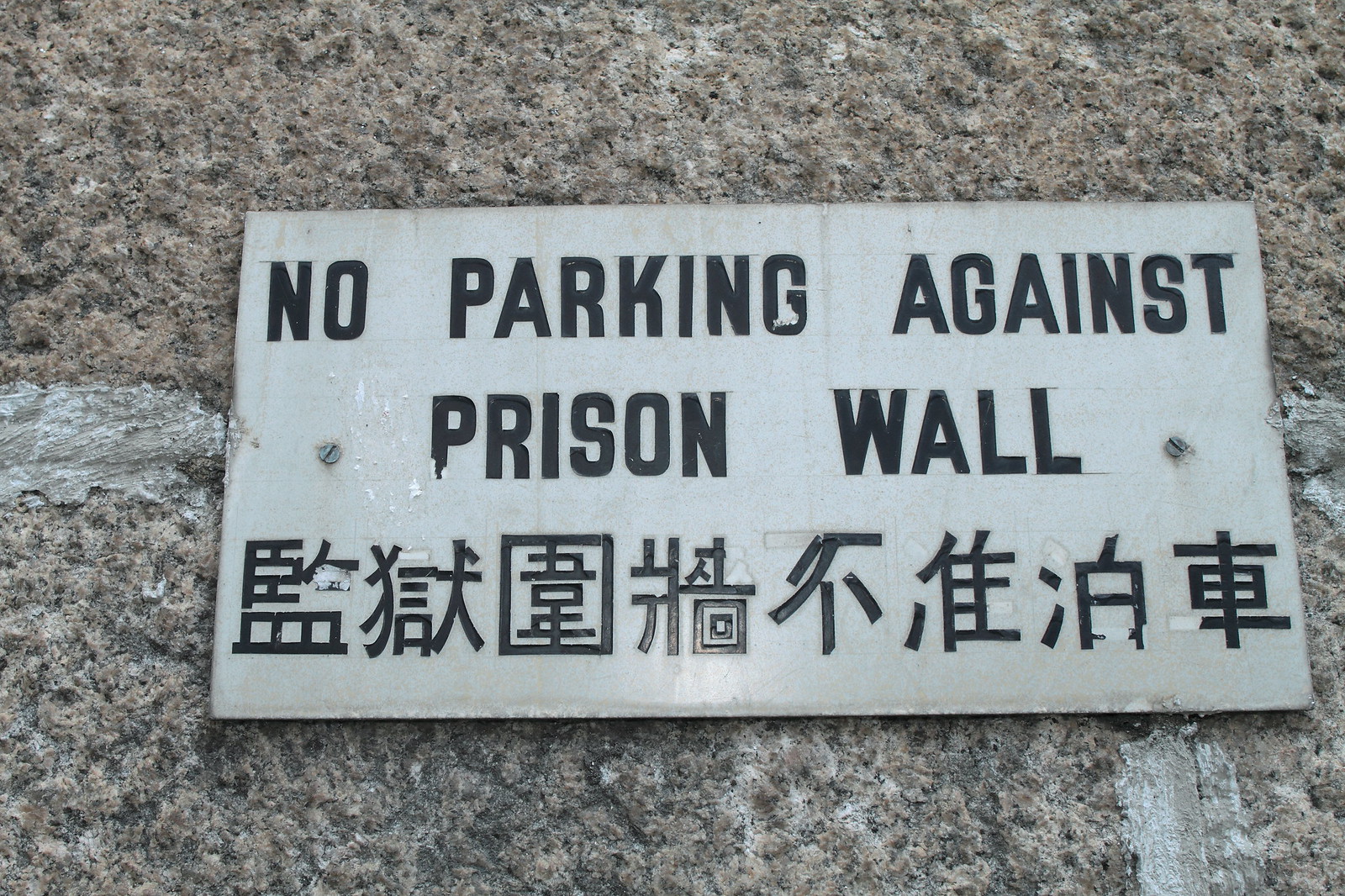A well-placed signboard is mounted on a rugged stone wall, adding to the historical ambiance of its setting. The signboard itself has a grey background and is prominently displayed on the wall. In bold, black capital letters, it clearly states: "NO PARKING AGAINST PRISON WALL". Below this, the same message is repeated in Chinese, accommodating bilingual readers. The backdrop of the sturdy stone wall suggests that it is part of a prison complex, reinforcing the seriousness of the warning.